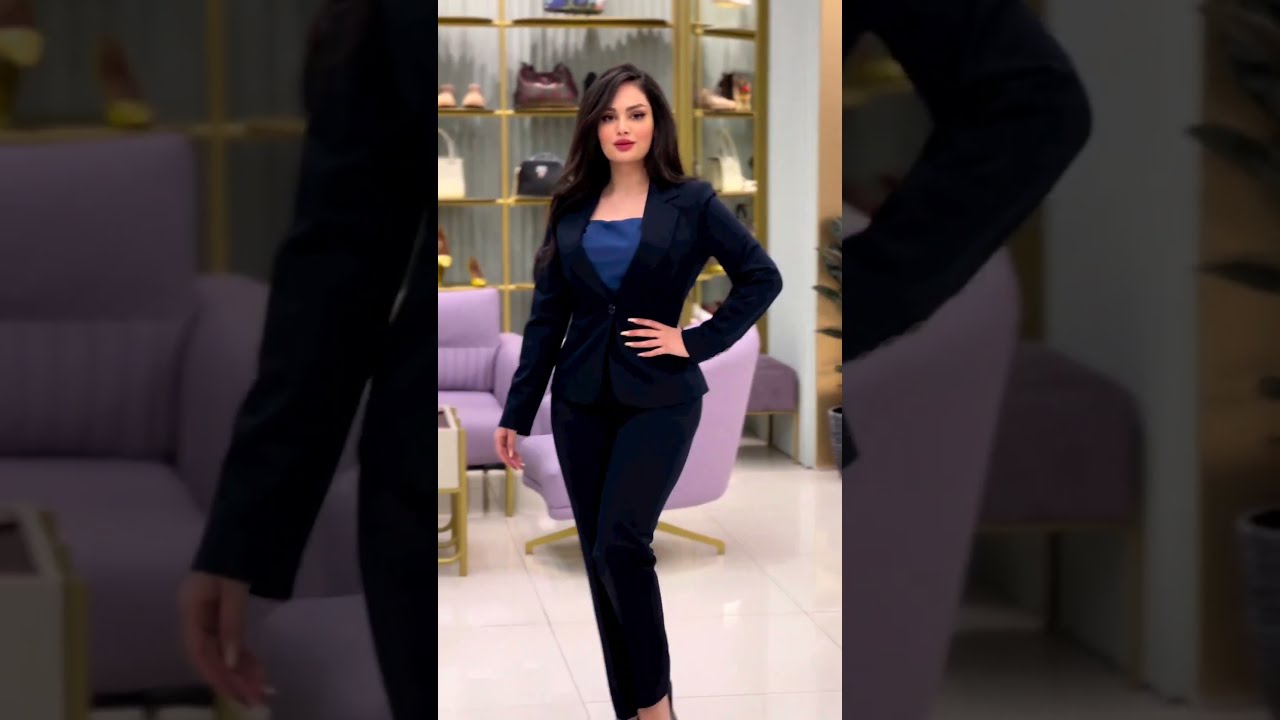In the center of the image stands an attractive, slim woman, possibly in her early 30s, with long black hair and striking red lips. She is posing confidently with her hand on her hip, dressed in a stylish black blazer and matching trousers, with a blue top underneath. The setting appears to be a salesroom for designer goods, showcasing a variety of handbags and shoes. The floor consists of large, shiny beige tiles that add to the room's bright and polished appearance. Behind the woman, there are two purple seating areas: one is a freestanding swivel chair, and the other appears to be a portion of a loveseat, separated by a white rectangular coffee table. Further in the background, a shelf adorned with mustard green frames displays numerous handbags, while other shelves feature an assortment of shoes, including tan, yellow, and brown high heels. The overall composition suggests a high-end, vibrant retail environment.